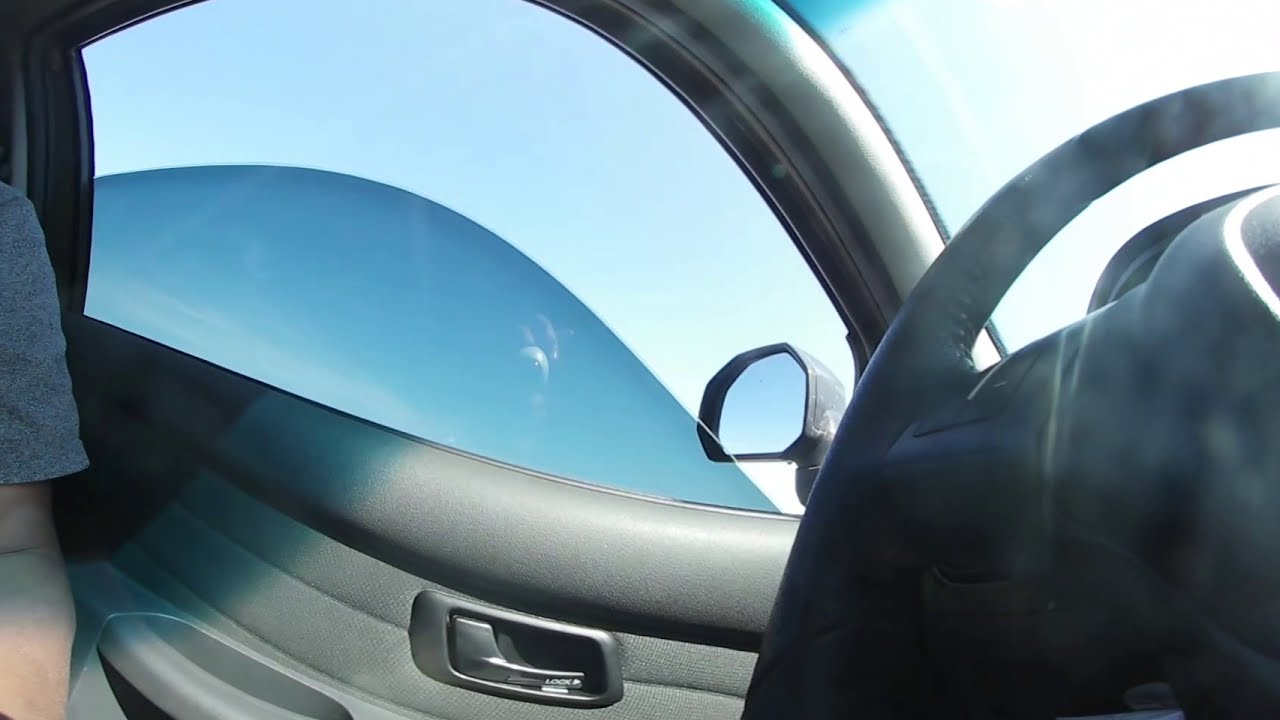The image captures a detailed view from inside a car. The gray interior is emphasized, showcasing the car door with its medium to light gray door handle and the partially opened window. The scene is lit by sunlight streaming through a mostly clear blue sky with a few misty clouds. A steering wheel, clothed in dark gray, occupies the right-hand side, while a side mirror reflects an indistinguishable shape that might be a dog. On the far left, part of a person, specifically an arm in a short-sleeved gray t-shirt, is visible. The windshield allows light to pour into the car, illuminating the gray tones within. The exterior environment is primarily serene blue sky, giving a sense of openness and calm.